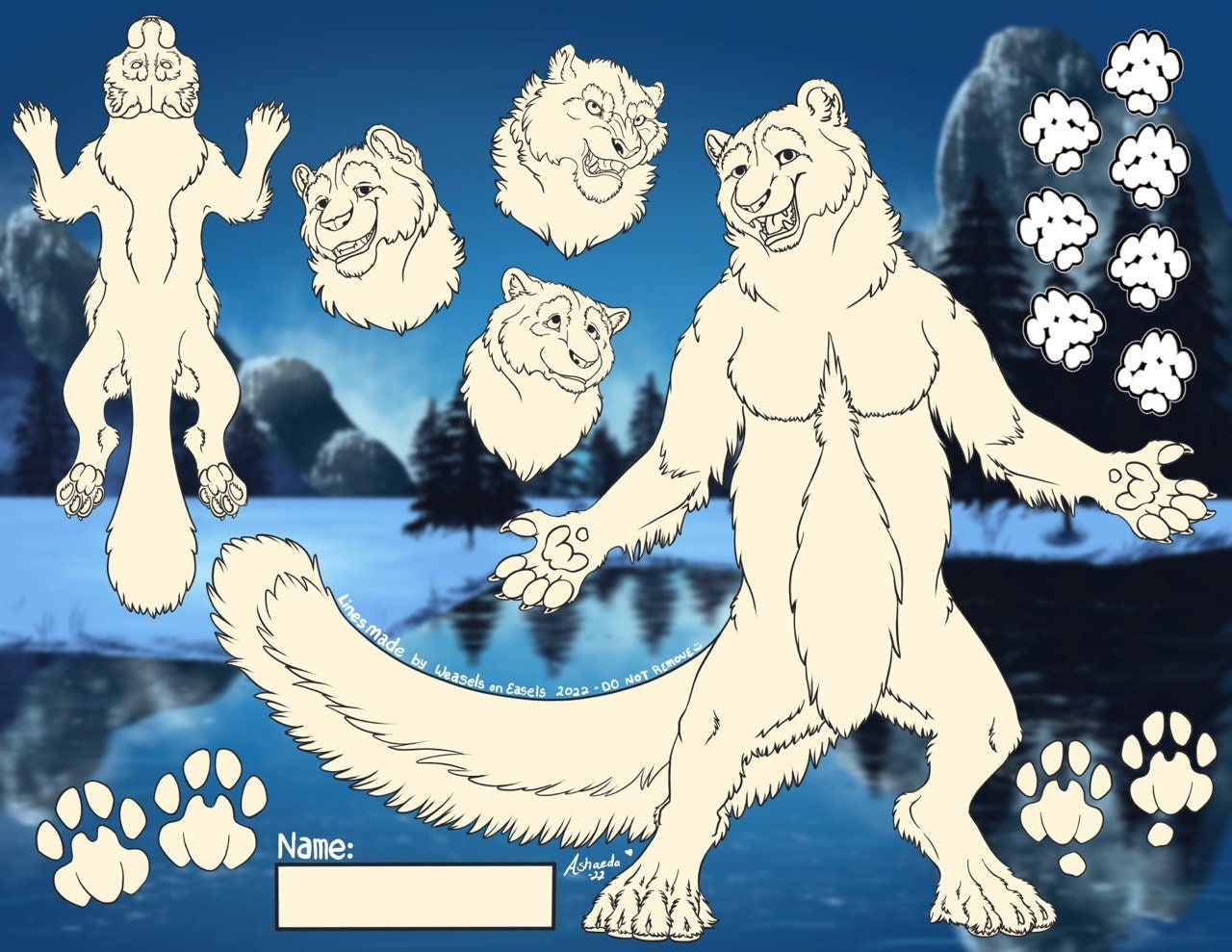This detailed image depicts a cartoonish, anthropomorphic creature, which could be a bear, leopard, lion, or even a snow leopard. The main figure stands upright on its hind legs on the right side, with its arms outstretched as if shrugging and its head tilted to the left, sporting a wide smile. A thick, furry tail emerges from behind it, trailing to the left side of the image. Surrounding this figure are numerous paw prints, and to the left, a series of close-up facial expressions showing the creature looking happy, angry, and confused. Additionally, there is a whimsical drawing of the creature flattened like a rug near the top left corner. All the illustrations are rendered in black and white, with bold outlines and white interiors. Further beneath the image, on the bottom left, is a designated area where a name can be written in. The image has a playful and slightly whimsical ambiance, enhanced by the phrase "lines made by weasels on easels 2022 - do not remove," perhaps hinting at the artwork being a fun, digital coloring activity. The background features what resembles an icy lake and glaciers, contributing to the predominantly white and pale blue aesthetic.